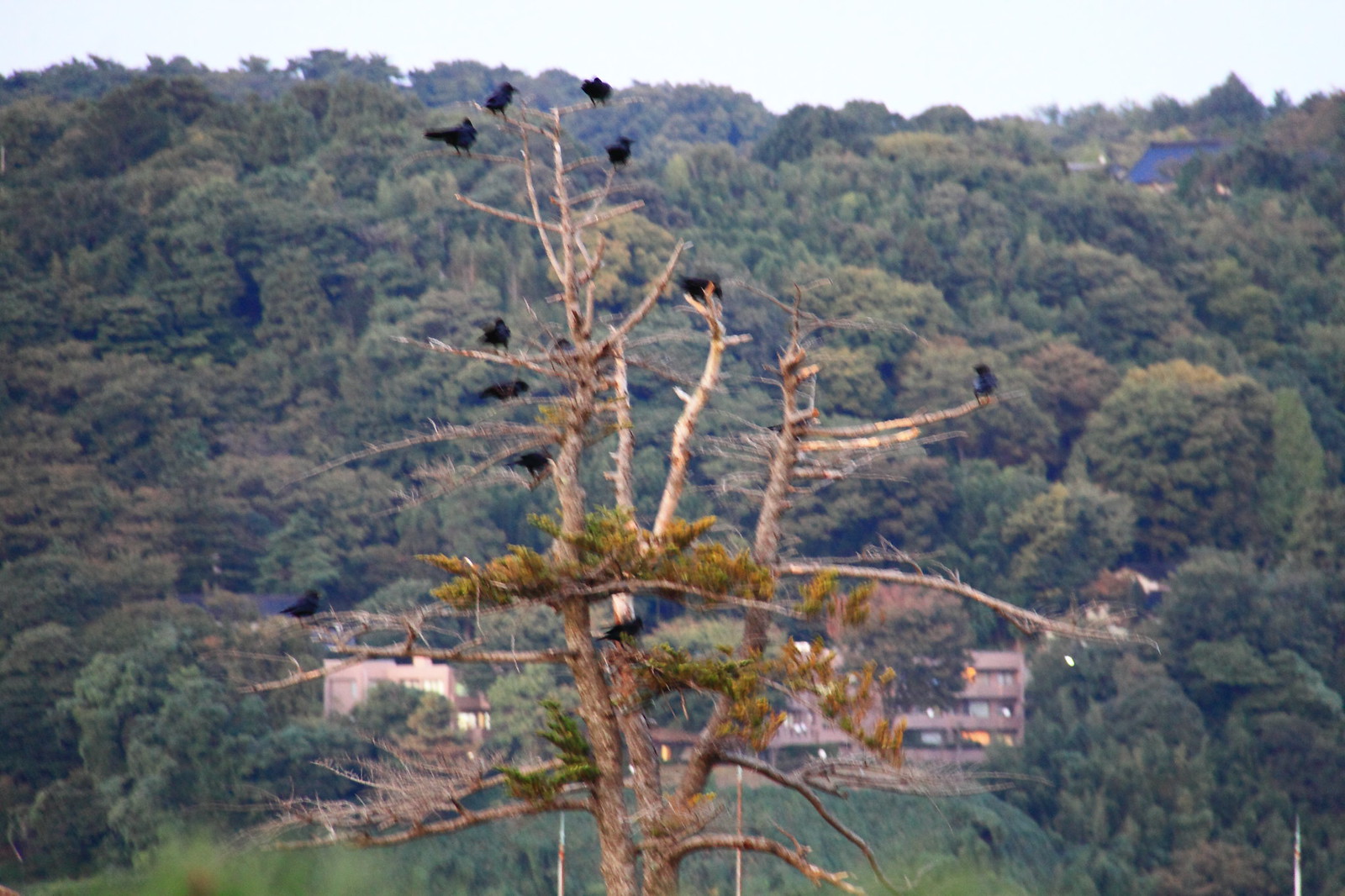The image captures a nearly bare tree with sparse leaves and needles, some of which are dark green and golden yellow, possibly indicating it's off-season or the tree is dying. Perched on its branches are ten black crows. The tree stands in sharp contrast to a lush, rolling background of green and seasonally changing yellow-brown trees. At the lower center of the background, partially obscured by trees, is a building with a red-brick exterior, possibly an apartment building with balconies and a large blue roof. The sky overhead is a consistent gray, suggesting an overcast, cloudy day without any visible text.